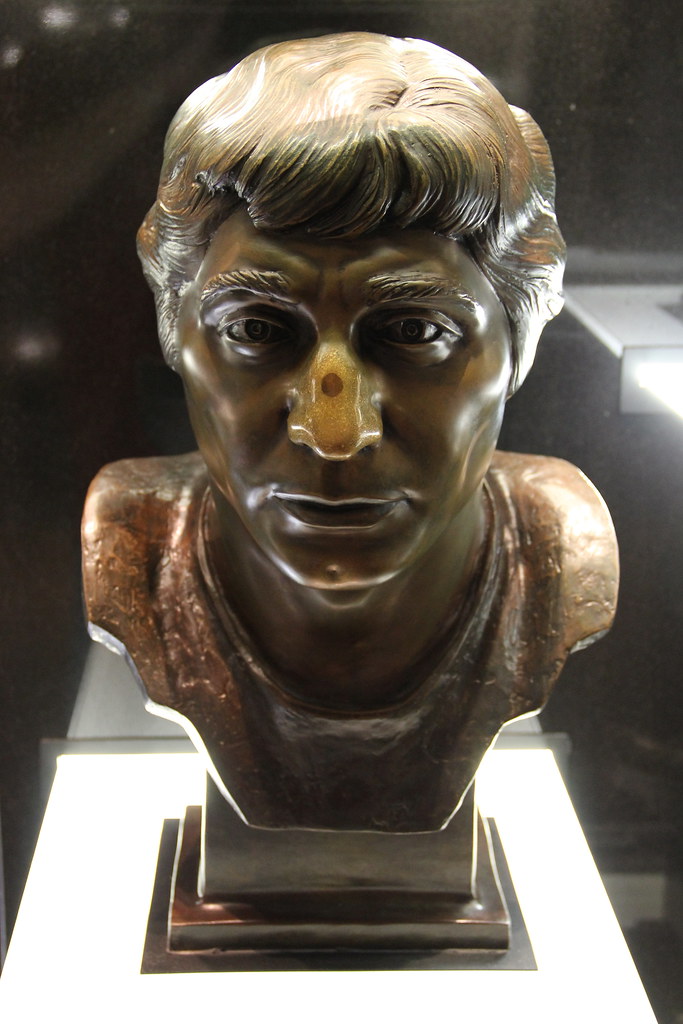In the image, a bronze or darkened bronze bust of a man sits prominently on a well-lit white pedestal, hinting at a museum or showcase setting. The bust, capturing the head and chest, portrays a male figure with a stern, staunch expression. His short, poofy hair is meticulously crafted, covering his ears while reflecting some of the surrounding lighting, casting whitish highlights. Notably, there is an off-color dot on his nose, suggesting some wear or an intentional feature. The background is non-distinct, with a brownish hue, sporadic light glares, and some vague shapes, including a silverish rectangular block. The absence of any identifiable markings or inscriptions on the base leaves the figure's identity open to interpretation, though he bears a resemblance to historical figures like Julius Caesar or a Roman general.